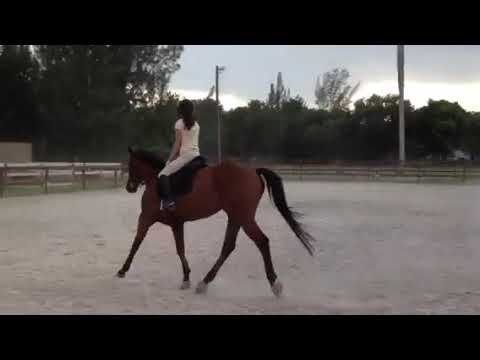In the image, a young woman is riding a bay horse with a dark brown coat and a sleek, long black tail. The woman, dressed in a white shirt and white riding breeches, rides in an English saddle and appears to be trotting the horse in a dusty arena. The arena, encircled by a wooden fence, has a sandy ground with no grass. Beyond the fence, trees with lush green leaves and silver-colored poles are visible under a heavily clouded, gray sky, suggesting an impending storm or early evening. The woman, whose face is not visible, is seen from behind, and she has mid-length black hair possibly covered by a black helmet. There are no other people or animals in the image.